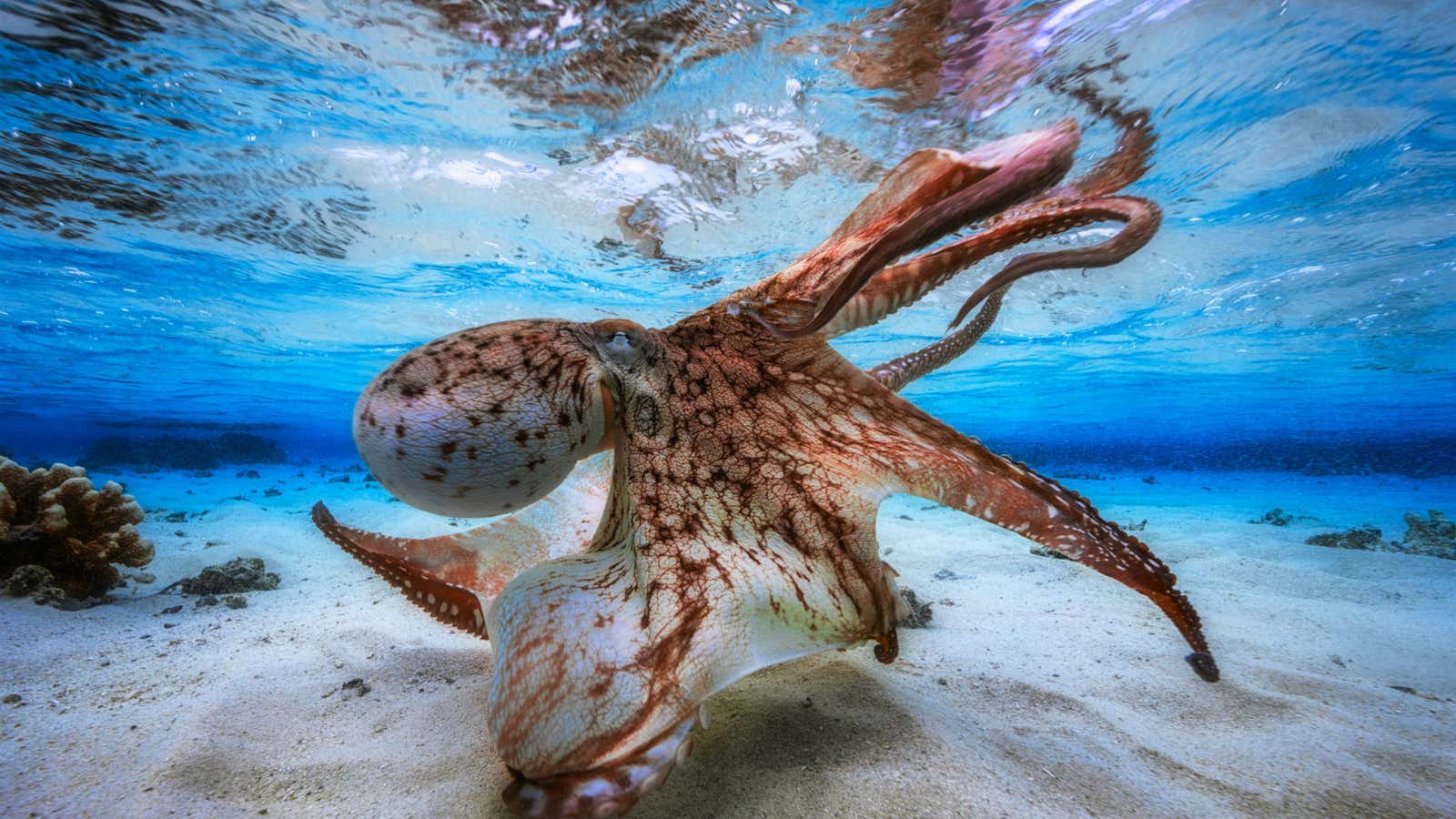This underwater photograph, taken in a landscape orientation, presents a striking view of a large, brown, and white-patterned octopus floating just above the sandy ocean floor. The octopus is prominently featured in the center, with its bulbous head facing the left side of the image. Its tentacles stretch out gracefully, with one extending towards the viewer and others fanning out towards the right. The background displays a beautifully clear blue sea, with light and dark blue gradients creating a sense of depth. There are ripples and reflections on the water's surface above, suggesting the octopus is in shallow water, possibly within 10 feet from the surface. The ocean floor below is composed of light yellowish-brown sand, interspersed with a few rocks visible in the upper left and center right of the image. The overall scene is a realistic portrayal of marine life, capturing the ethereal beauty of the underwater world.